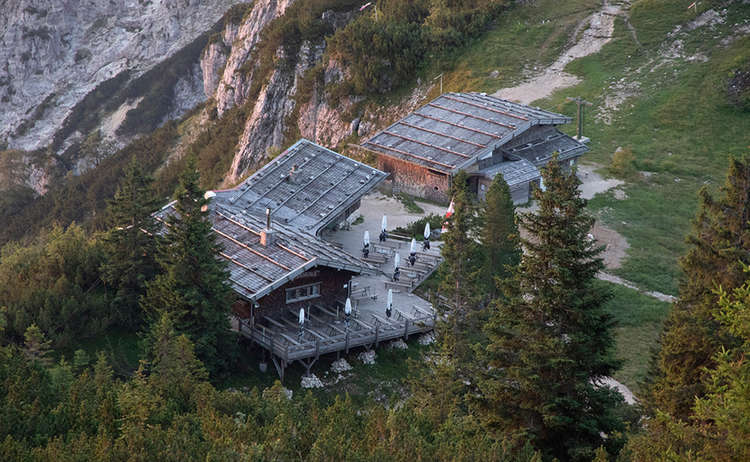The photograph depicts an advanced, sizable building complex set against a rugged, mountainous backdrop. The scene includes two main structures situated in the center of the frame, appearing to be nestled on the edge of a steep cliff or drop-off with uneven gray rocks visible, indicating the challenging terrain. The buildings are surrounded by a mix of hilly areas and densely packed evergreen trees, contributing to the natural, secluded atmosphere. 

The larger structure on the left, which resembles a resort or bungalow, features a hipped, slanted roof with linear patterns and a wrap-around porch furnished with tables and folded white umbrellas. This building exudes an inviting, yet serene appearance with its open front area and pathways. Across from it, on the right, stands a smaller structure also with a hipped roof, accompanied by what looks like a shed, possibly for vehicle storage. 

In front of the buildings, a path meanders through a grassy area, accentuated by strategically placed lights that guide the way. The right side of the image reveals several tall evergreen trees and a road or path leading towards the building, emphasizing the accessibility yet remote feel of the location. All these elements together create a vivid, detailed portrayal of this picturesque, cliffside retreat.